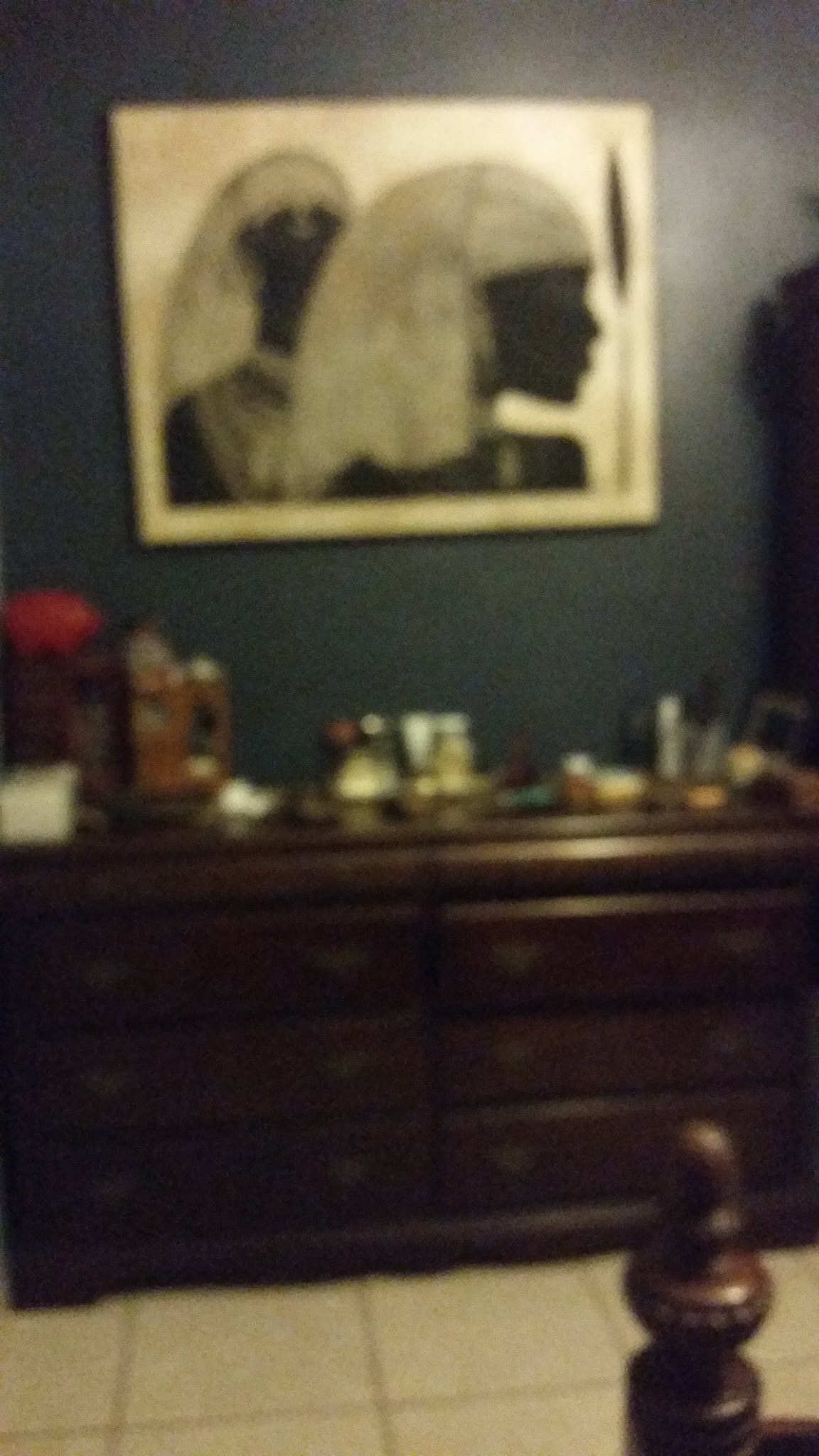The blurry photograph captures a bedroom featuring a dark brown dresser set against a dark blue or green wall, with a light tan or beige tiled floor. Central to the image is a distinctive black and white piece of art or illustration hanging on the wall. This artwork showcases two figures adorned in Egyptian headdresses, one figure looking left and the other looking straight ahead, possibly accompanied by a spear-like element on the right side of the image. The dresser beneath the artwork is cluttered with various indistinguishable items, including what appears to be red flowers. Although taken with a personal camera, the photo’s lack of sharpness makes finer details unclear, but the dark, moody tones of the room are evident.